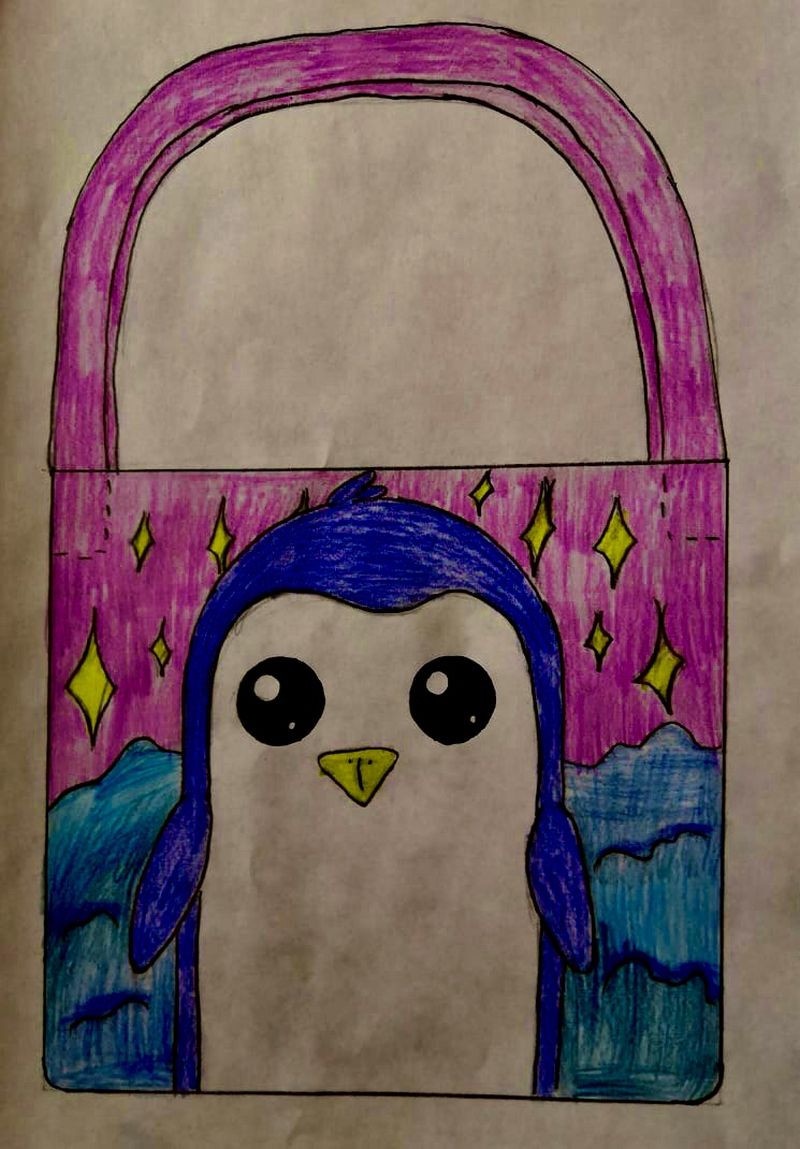This detailed drawing depicts a hand-crafted image of a purple penguin tote bag or purse, rendered on what appears to be a piece of white construction paper. The top portion of the bag, along with the handles, is colored in a uniform purple shade, adorned with yellow diamond patterns. Dominating the center of the tote is a large, adorable penguin characterized by its round, black reflective eyes, a yellow triangular beak with a "T" marked on it, and blue feathering accentuating its arms and head. Below the penguin are large blue formations, which may represent mountains or waves of water. The background also features additional elements like squiggly lines, possibly highlighting more detailed aspects such as water or ice, and small stars scattered throughout the drawing, adding to the whimsical and endearing nature of the illustration.